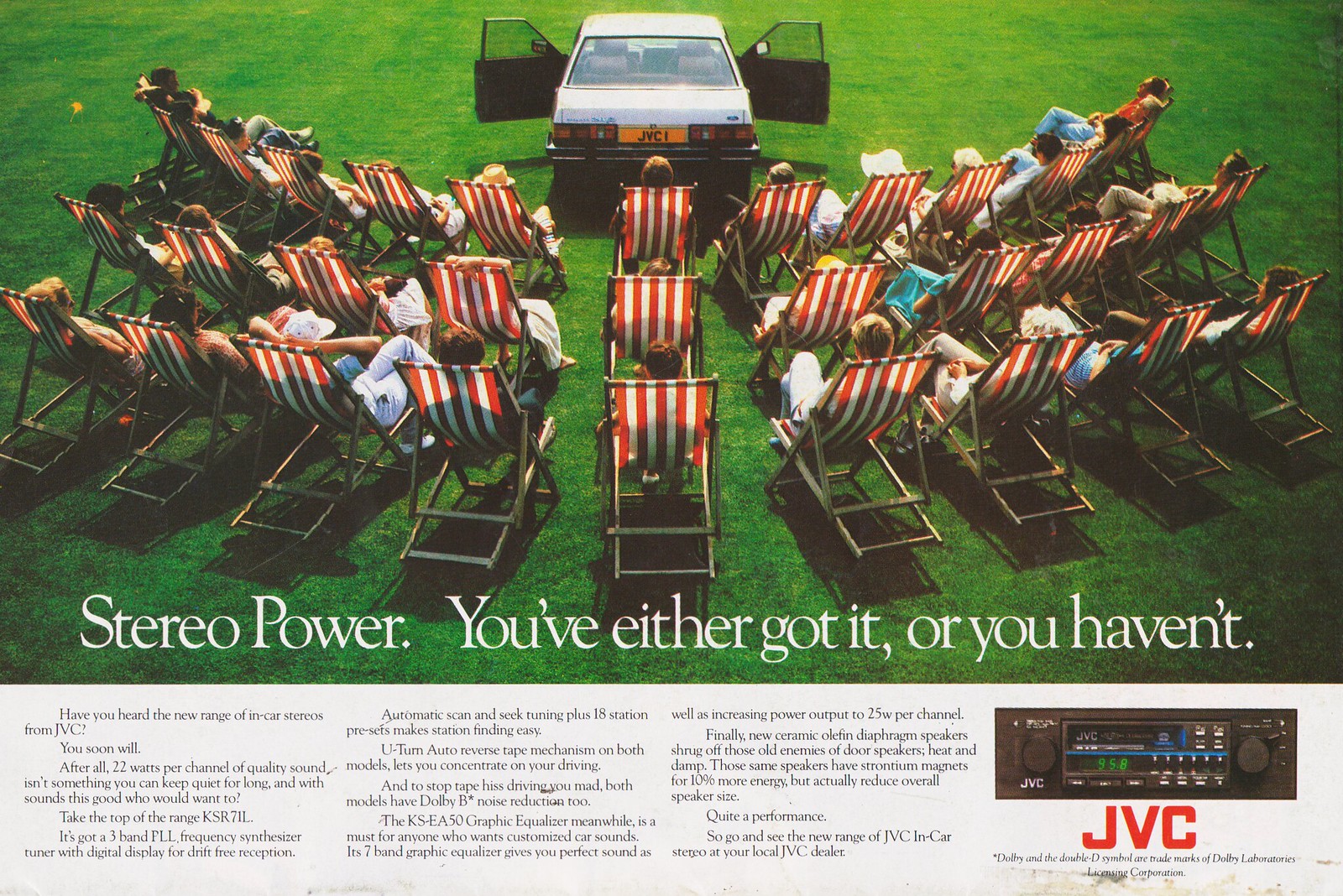The advertisement showcases a vibrant summer scene with a car in the foreground, its doors wide open, suggesting the source of music. In front of the car, an open green field is dotted with rows of lawn chairs, which have red and white or orange and white striped fabric. The people lounging in the chairs, dressed in casual summer attire, appear deeply absorbed in the music emanating from the JVC car stereo. They sit comfortably, creating a semicircle or three rows, reinforcing the communal enjoyment of the stereo's sound. Prominently displayed at the bottom of the ad is the slogan in bold text: "Stereo Power, you've either got it or you haven't." Additionally, in the bottom right corner, a small image of the car stereo is accompanied by the brand name "JVC" in red lettering. Below this, there is a block of small, detailed text describing the stereo's features, though it is not easily readable. This evocative scene emphasizes the superior sound quality and communal joy provided by JVC's car stereo, appealing to potential customers' desire for exceptional in-car audio experiences.